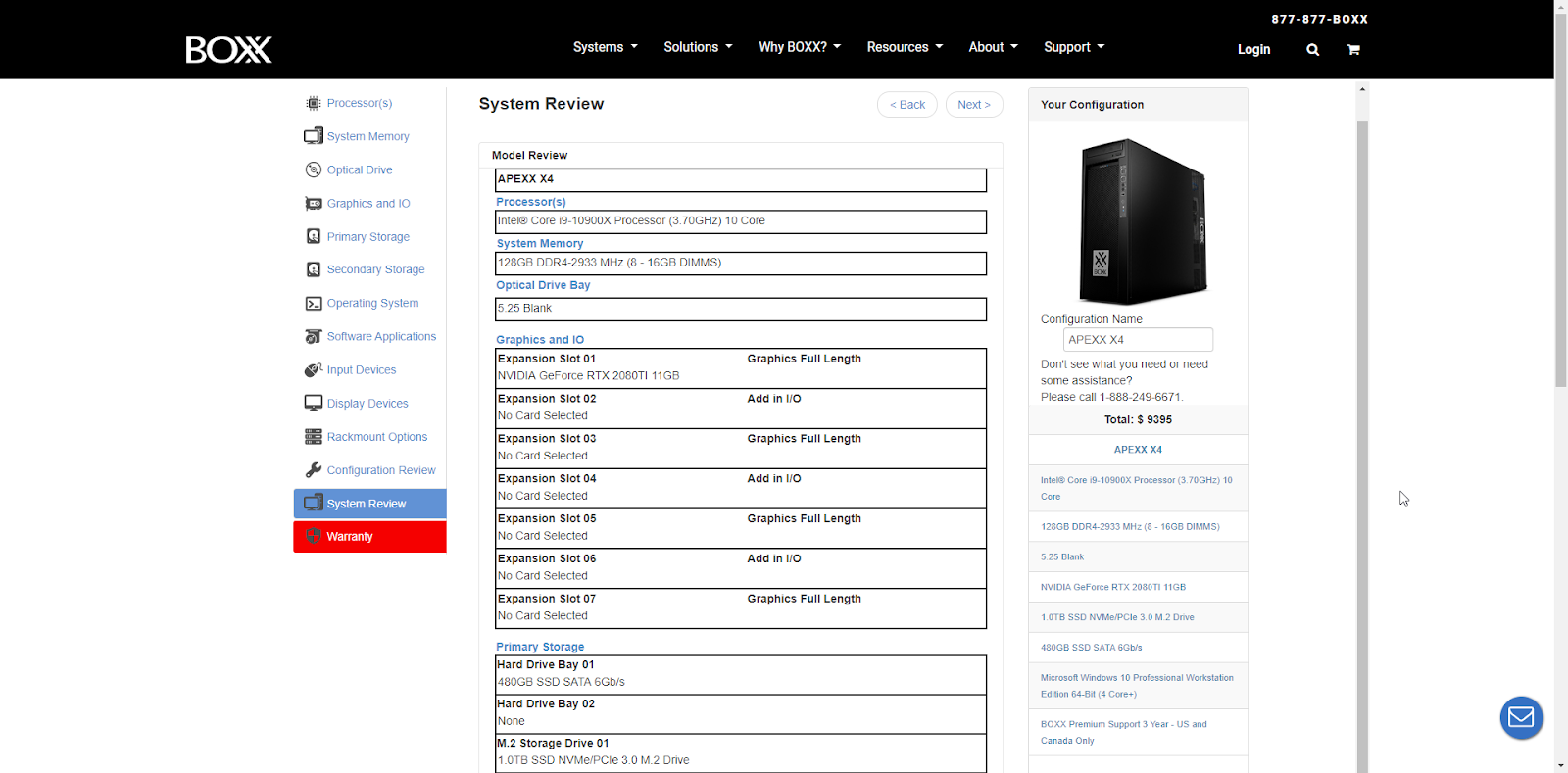The website's interface features a prominent black menu bar on the left-hand side, along with a matching black navigation bar at the top. The top bar displays the company logo, "BoxBOXXX," at the leftmost part. To its right are several menu options organized sequentially: System, Solutions, YBox, Resources, About, and Support. Further right, users will find icons for logging in, searching using a magnifying glass icon, and shopping via a shopping cart icon. Above these icons, a contact phone number is clearly displayed, likely for customer service inquiries.

Below this primary navigation, the main content area lays against a clean, white background. On the left side, filtering options are available, although the font size is quite small. There are 12 distinct filter categories listed. Beneath these filters are two buttons: a blue "System Review" button and a red "Warranty" button.

To the right of the filtering section and buttons, there's a detailed "System Review" area featuring several sections or fields for user interaction. Adjacent to this, a section labeled "Your Configuration" includes a photograph of a desktop computer with a list of specifications and options beneath it. These options offer detailed information about the desktop computer, though the small font makes it difficult to read.

In the lower right-hand corner of the page, there is a small blue button with a mail icon, presumably for users to contact customer support via email. This comprehensive layout ensures that users can easily navigate through various system configurations, access support, and review product details efficiently.